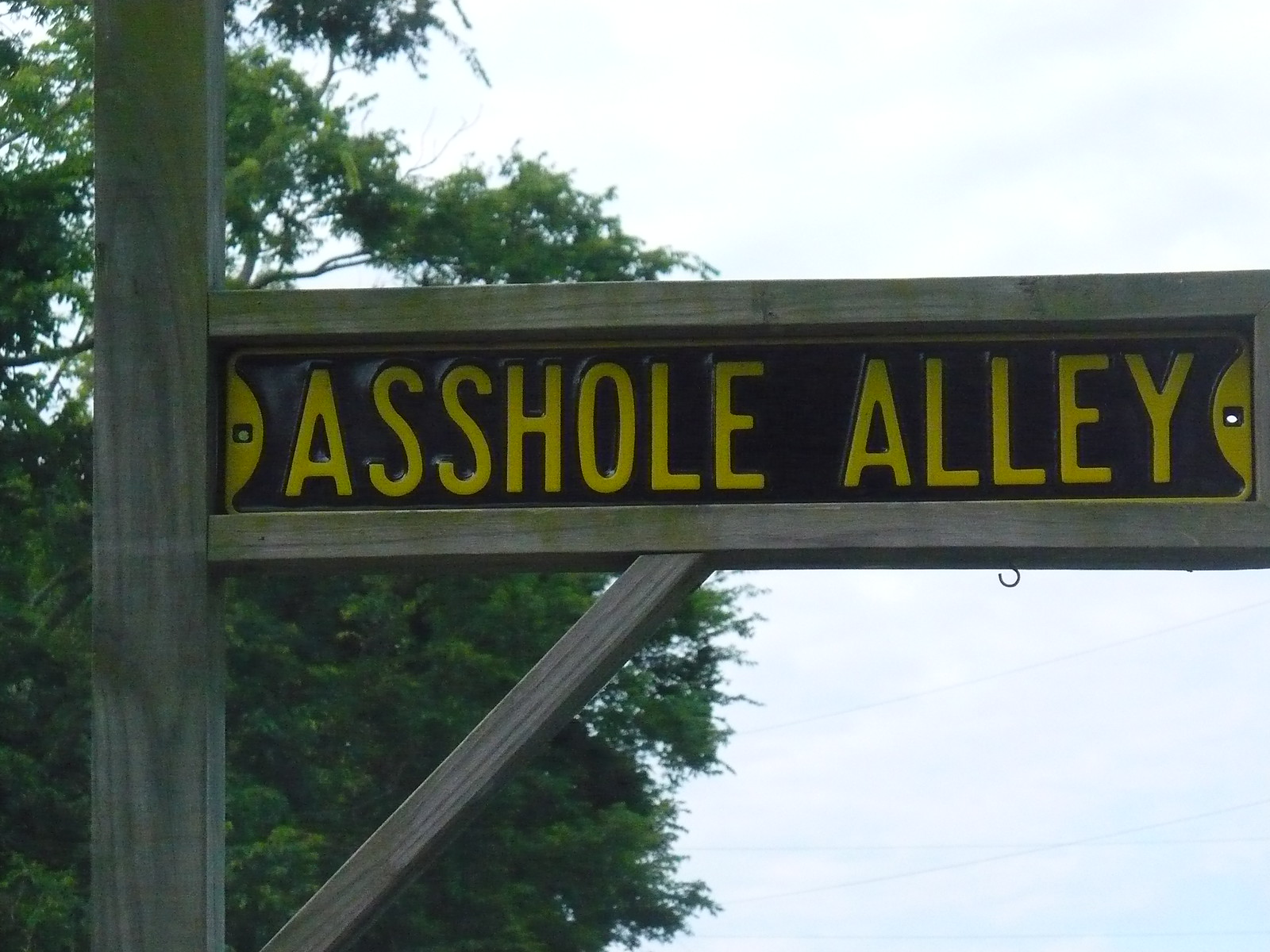The image is a color photograph of a sign titled "Asshole Alley" mounted on a wooden post. The sign features bold, yellow, capital sans serif letters on a black background, reminiscent of an old-fashioned license plate with embossed or punched text. The wooden frame around the sign appears to be made from pressure-treated 2x4s, with additional angled 2x4s for structural support. The post itself is a sturdy 4x4, also made from pressure-treated wood. The photograph was taken during the day, capturing a cloudy and hazy sky along with some trees in the background, indicating the photo is angled upwards. The overall structure and custom nature of the sign suggest it is more likely a whimsical, personal creation rather than an official street sign.